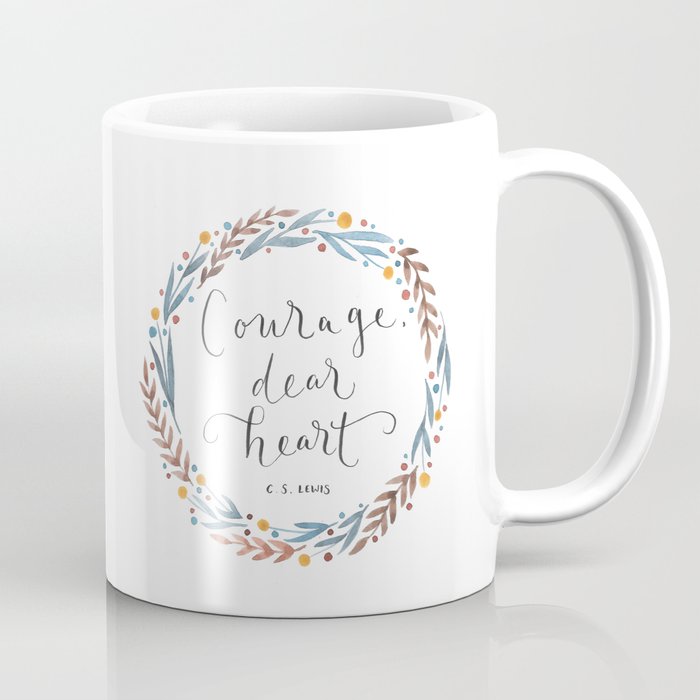This photograph features a white coffee mug on a shiny white table with a white wall as the backdrop. The mug, with its large handle positioned to the right, casts a subtle shadow on the table. Central to the mug’s design is a circular wreath made of laurel-like leaves in shades of light gray and tan, with hints of yellow, purple, and gray giving it a Romanesque feel. Interspersed within this intricate wreath pattern are small golden dots, complemented by tinier magenta and blue accents throughout, adding a delicate decorative touch. In the center of the wreath is a cursive inscription that reads "Courage," "Dear," "Heart" on separate lines, attributed underneath to C.S. Lewis in a smaller, Times New Roman-like font. This elegant and inspirational quote by the famous author is stylishly presented, suggesting the mug might be part of a product line aimed at conveying motivation and aesthetic appeal.